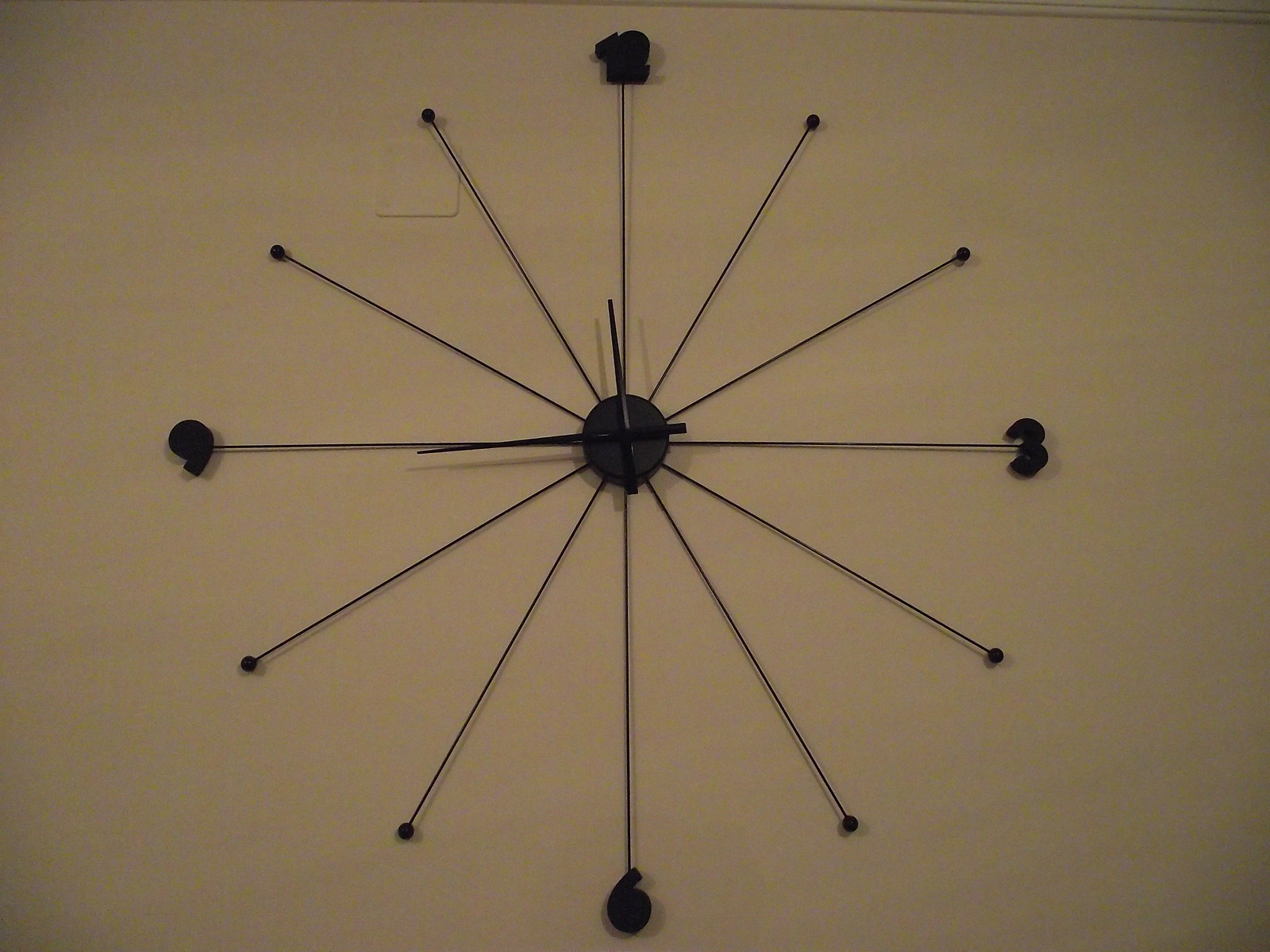The image depicts a large, minimalist clock mounted on a white wall, illuminated by soft room lighting. The clock features 12 thin, black lines radiating from a central black circle, each ending in a small dot corresponding to the hour marks. The only visible numbers are 12 at the top, 3 on the right, 6 at the bottom, and 9 on the left. The clock's hands, which appear to be black, indicate a time of quarter to twelve, with the hour hand pointing at 12 and the minute hand at 9. The overall design gives an impression of a floating system of lines, with no traditional clock base or background.